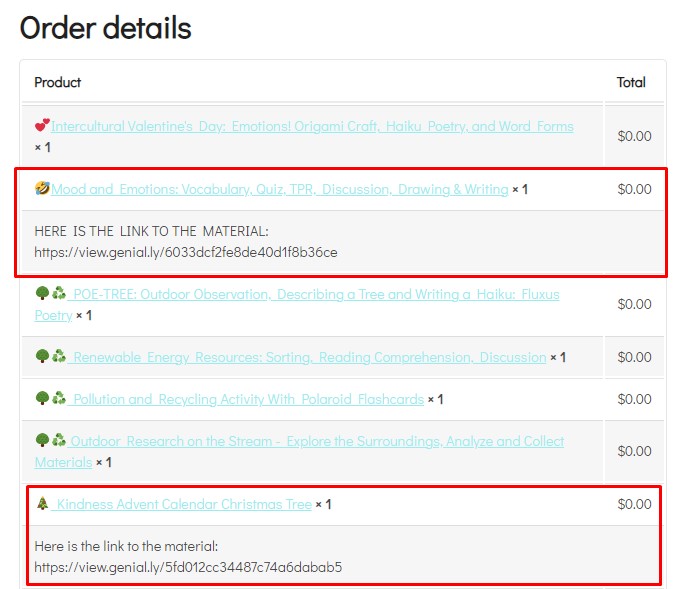The image displays an order details page with a clean layout emphasizing the different sections of the order. At the top of the page, the heading "Order Details" is printed in bold black font. Below it, a white rectangle highlights the headings "Product" and "Total." 

As you scroll down, there's an interactive section featuring various items. One of the highlighted items is "Intercultural Valentine's Day Emotions Origami Craft Haiku Poetry and Word Forms," which is listed at a total of zero dollars. Adjacent to this, there is an area titled "Mood and Emotions Vocabulary Quiz TPR Discussion Drawing and Writing," which also costs zero dollars and includes a clickable HTTPS link to the material. This entire section, starting from "Mood and Emotions Vocabulary Quiz" down to the HTTPS link, is bordered by a large red rectangle.

At the bottom of the page, another item listed is the "Kindness Advent Calendar Christmas Tree," marked as one unit with a total cost of zero dollars. This item also includes a link to the material, presented as an HTTPS URL. 

Additionally, there are three or four other sections on the page, all displaying a cost of zero dollars. Some sections feature icons like a recycling symbol or a green tree, adding a visual variety to the otherwise text-heavy content.